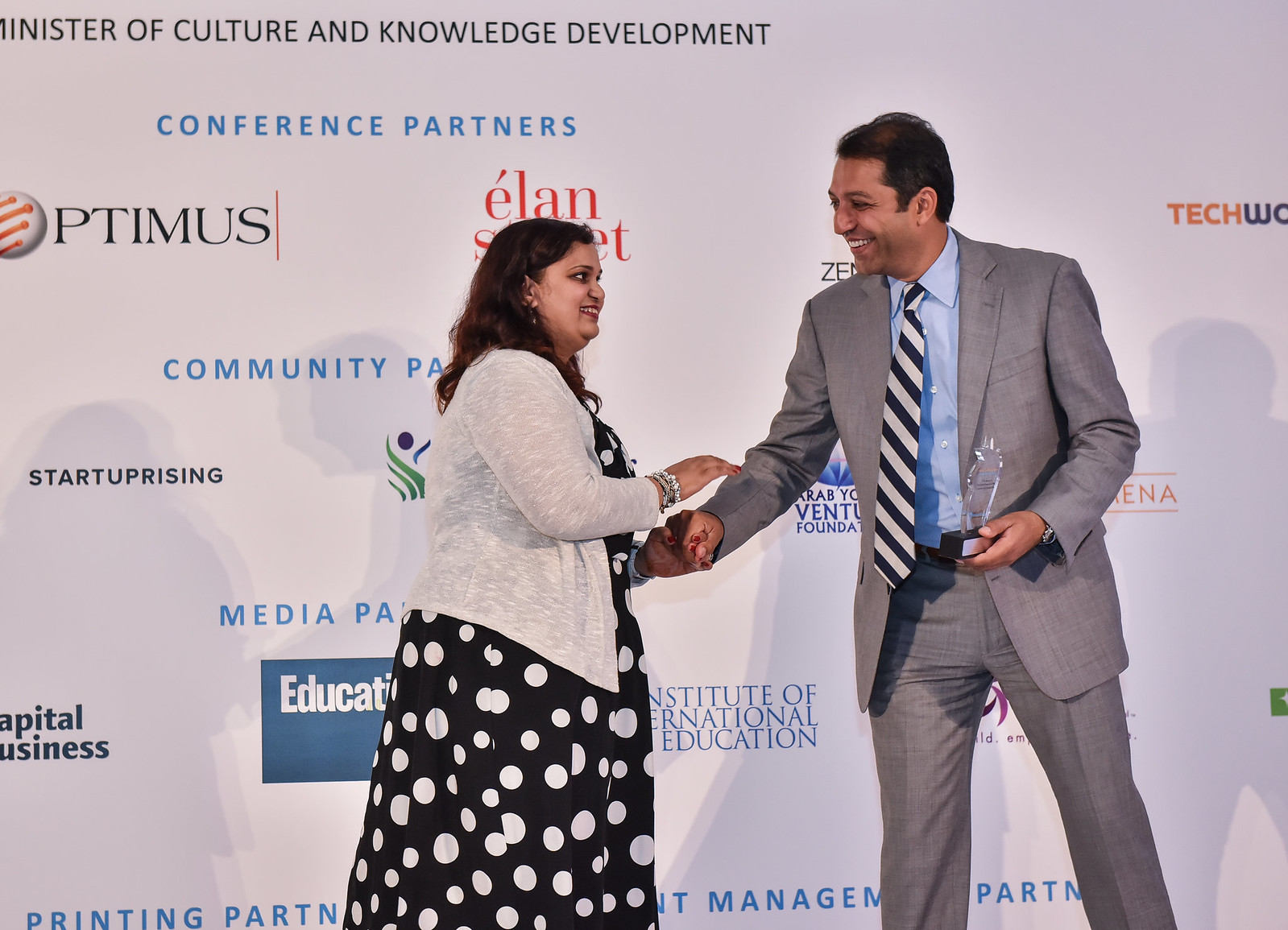In this photograph set in a professional environment, two individuals, both of Indian descent, are captured in mid-handshake, smiling and engaged with each other. The woman on the left is wearing a black dress adorned with white polka dots, complemented by a white sweater. She has long black hair and stands confidently as she engages with the man on the right. He is dressed in a gray suit paired with a black and white striped necktie and a light blue collared dress shirt. He sports a black wristwatch on his left arm and is holding a clear glass plaque or trophy in his left hand.

The backdrop is a white wall featuring various company logos and text. Prominently displayed at the top left are the words "Minister of Culture and Knowledge Development" followed by "Conference Partners" in blue. Beneath that, logos for companies such as Optimus, Startup Rising, and Capital Business are visible. The overall setting and the presence of the award suggest that this image was taken at an award ceremony or a similar formal event.